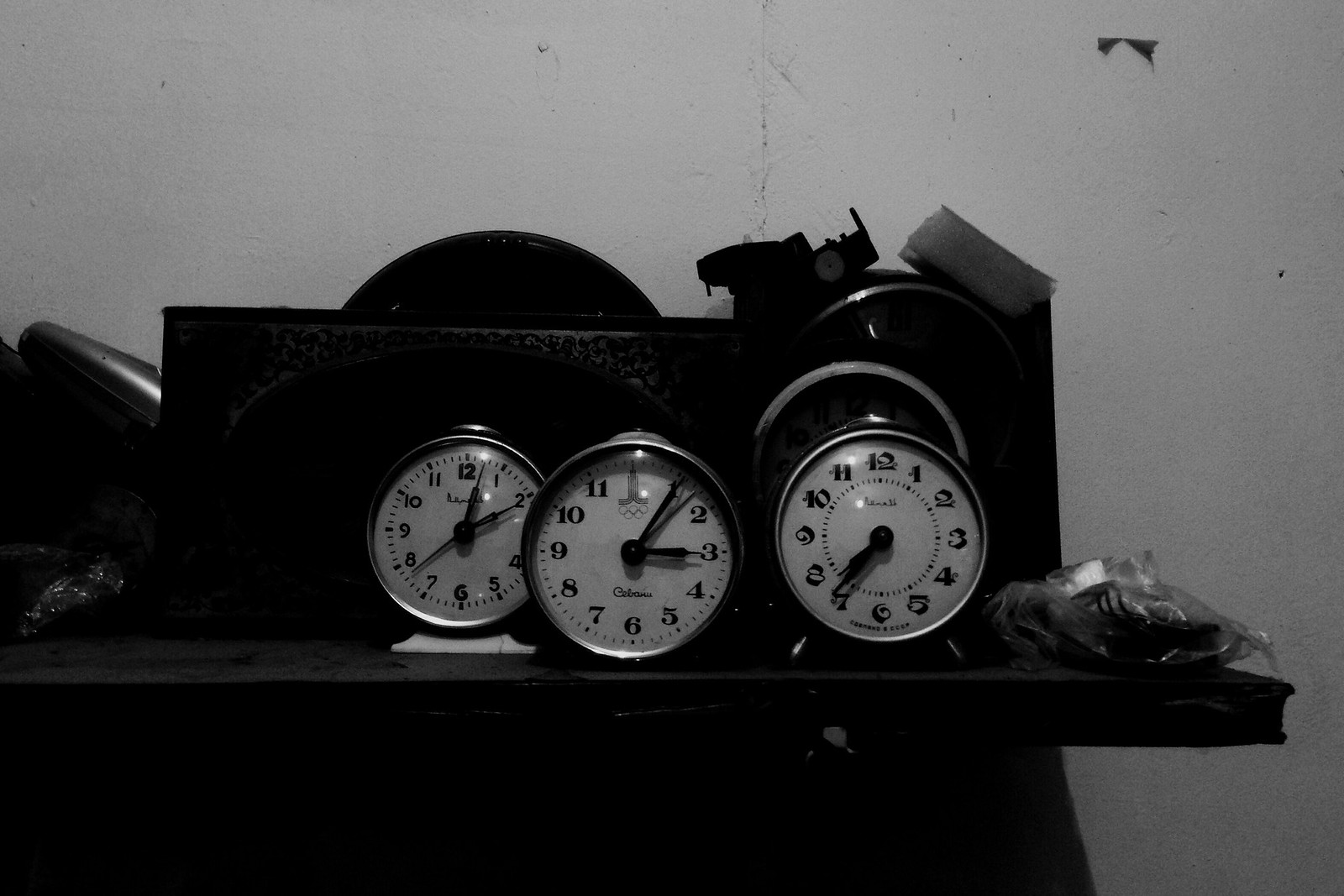This horizontally rectangular, dimly lit black and white photograph captures a trio of vintage style clocks placed on a dark shelf, all with circular faces rimmed in silver and black. Each clock has a white face with black numbers and hands, and they display different times: the left clock shows 2:02, the middle clock shows 3:05, and the right clock shows 7:36. The glass faces of the clocks reflect light from above or behind the photographer, causing a slight glare. Behind the clocks is a mysterious black box topped with various indistinguishable objects, including a plastic-wrapped item on the right. The backdrop features a grayish white wall due to the black and white nature of the photo, which adds to the vintage and somewhat blurry feel of the image, rendering the details in the background less distinct.